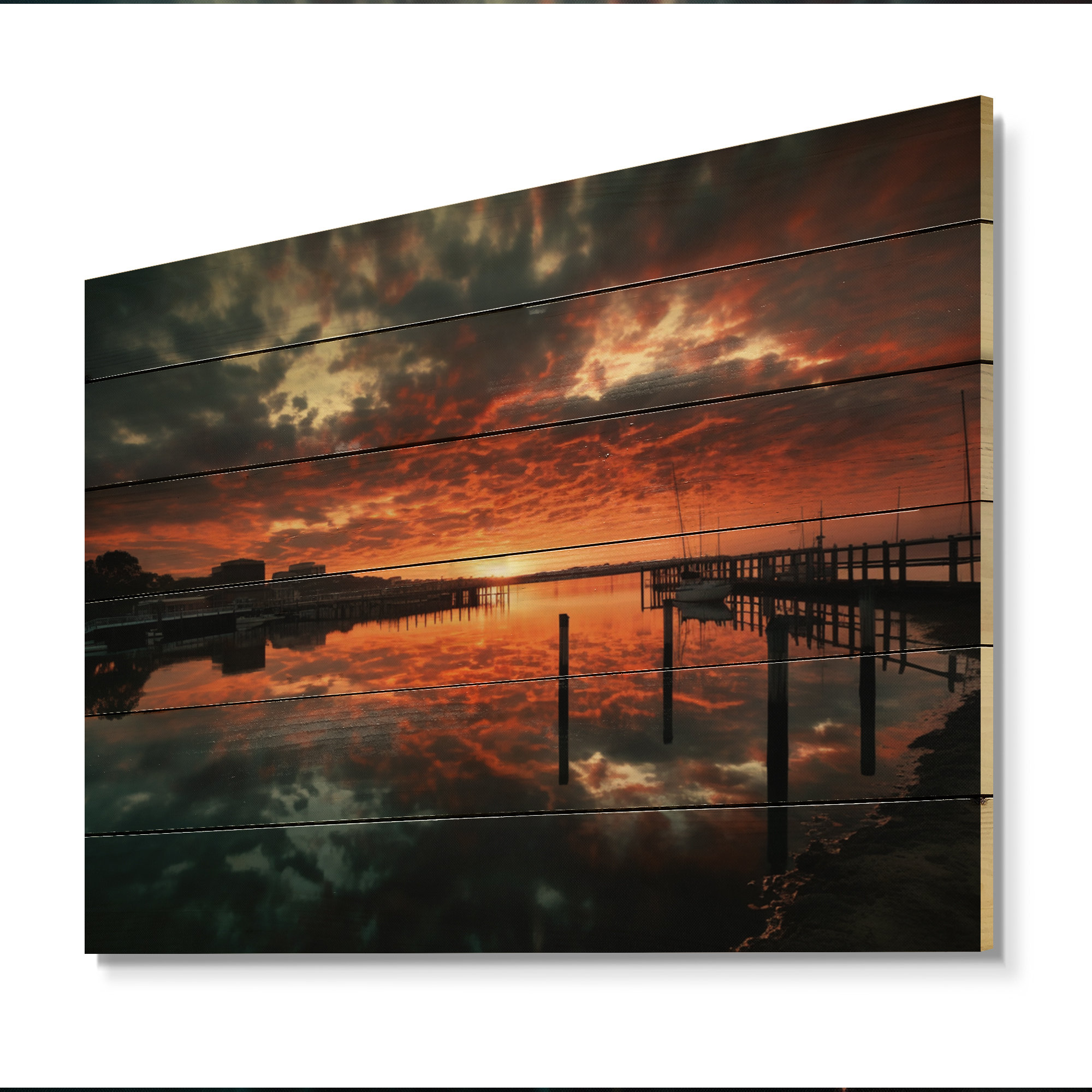This artwork, presented on six wooden plank boards, features a mesmerizing sunset scene. The planks are vertically aligned and arranged such that they form a cohesive image without a frame, ideal for wall display. Dominated by vibrant oranges, reds, and blacks, the top half of the artwork captures a sky painted with dark, puffy clouds tinged with a striking orange and black hue. The setting sun, centrally positioned, radiates light through the clouds, casting a warm glow over the scene.

Below, the bottom half consists of a reflection of the dramatic sky in the water, split neatly by the planks, with the far-left side showcasing dark green water transitioning to a darker shore on the bottom right. Subtle details like docks and muted buildings can be discerned on the left side of the image, contributing to the overall depth and ambiance without distracting from the main focus on the sky and its reflection.

Highlighted by thin black lines bordering the top and bottom edges, the artwork's unique composition ensures that the viewer’s attention gravitates towards the glowing sky and its captivating mirrored reflection in the water below. This dual focus creates a seamless, almost surreal visual effect, making it a truly stunning piece.